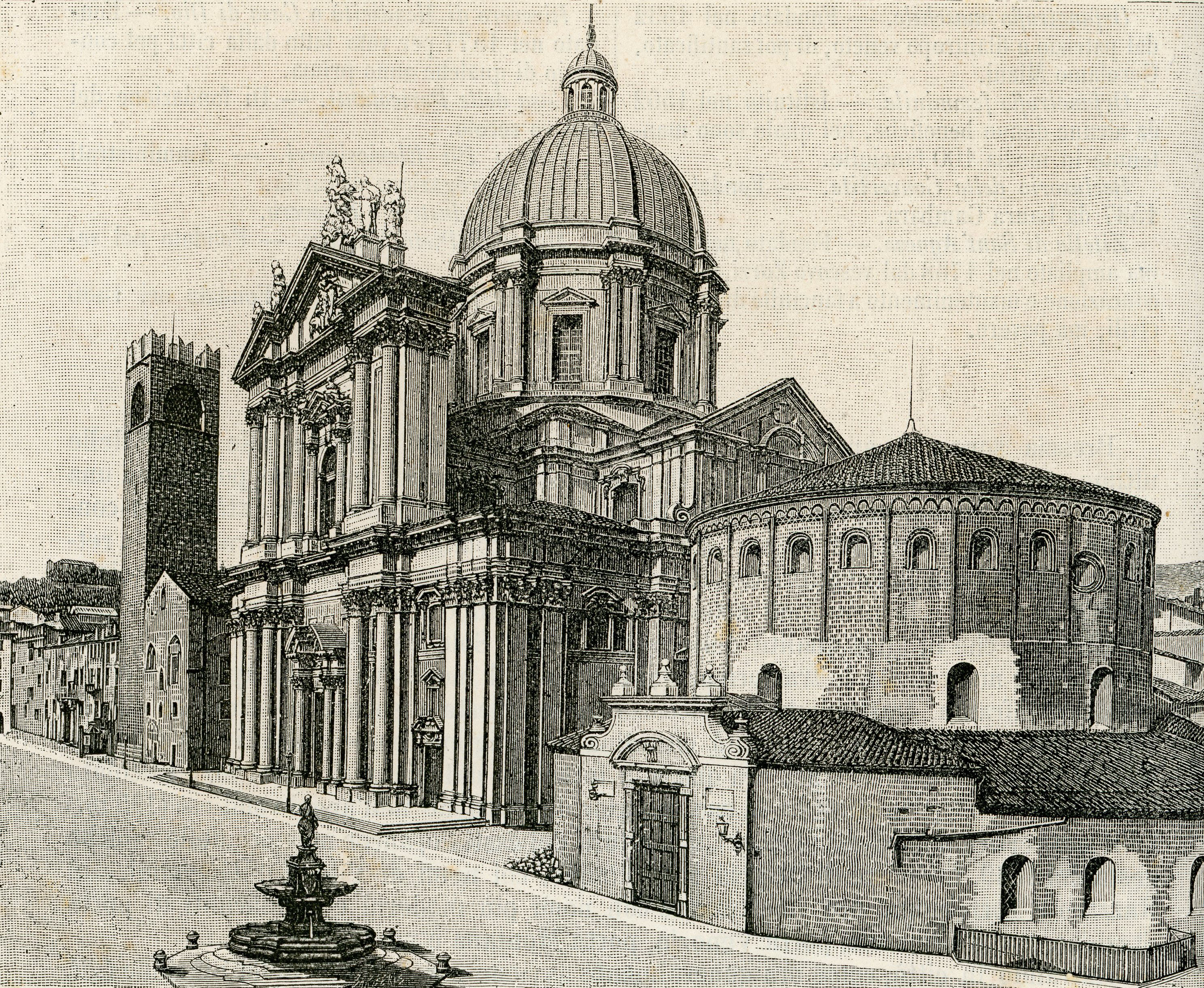This image is a meticulously detailed pen and ink sketch on gray parchment or paper, depicting a cluster of buildings that form a religious complex, set within an old European city. At the center is a prominent cathedral characterized by numerous intricate designs, tall columns, and stone-like statues resembling Renaissance art. To the left of the cathedral stands another striking structure, likely a church, marked by a towering bell tower. Adjacent to this church is a smaller yet notable building with a rounded area on top, supporting a dark dome and antenna, and featuring a discernible wooden door. The image also captures a cobblestone sidewalk and a fountain with a figure atop it, positioned in the foreground. The scene is brought to life with meticulous black and white detailing, illustrating a serene and historic urban atmosphere.